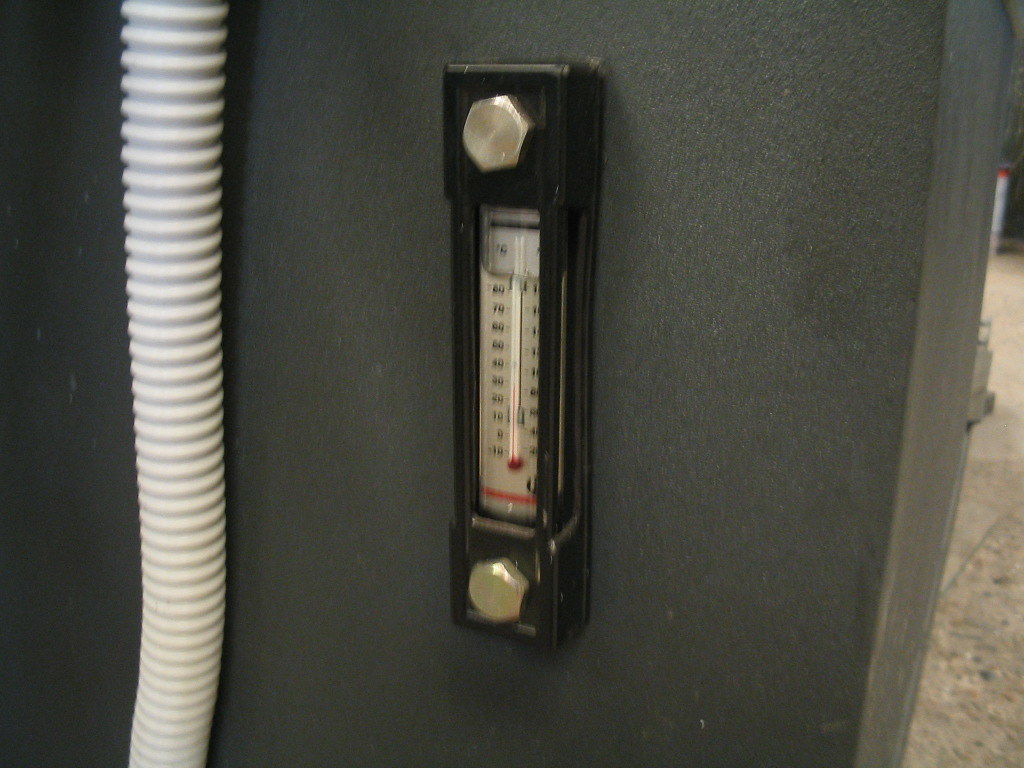The image depicts a wooden thermometer mounted on a gray wall. The photograph captures the corner of the wall, with one side extending to the left and the other side subtly receding into the background. The thermometer itself is crafted from a thick piece of wood, characterized by its tall and narrow structure. It features a prominent, six-sided silver bolt at both the top and bottom.

Central to the wooden frame is a white temperature gauge, accentuated with red stripes at both ends. The gauge includes a long tube containing mercury, culminating in a small round bulb at the bottom. Adjacent to the thermometer, a white plastic hose runs vertically along the wall. 

In the background, a small section of what appears to be a tan tile or presswood floor is visible, alongside some indistinct boxes occupying the lower right corner of the image. The wall and the objects within the frame gradually converge, eventually disappearing out of the shot at the top.